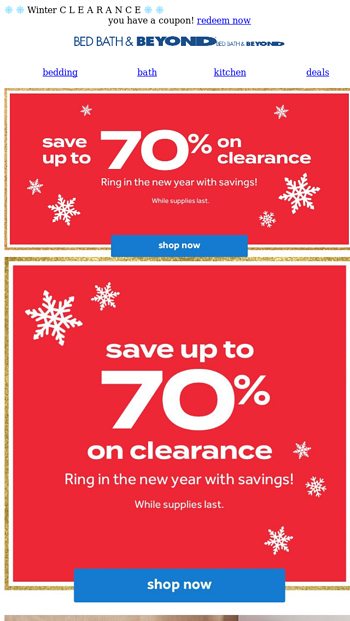This festive red advertisement is adorned with white snowflakes and features bold, white letters and elegant gold trim around its distinct sections. The ad is structured with a smaller red rectangular box at the top and a larger red square box at the bottom, both highlighted with glittering gold borders.

The red rectangular box contains six snowflakes of varying sizes and displays the message: "Save up to 70% on clearance. Ring in the new year with savings while supplies last." Directly beneath this box, nestled between it and the larger box, is a blue "Shop Now" button inviting immediate engagement.

The larger red square box, also embellished with gold trim and five snowflakes of different sizes, echoes the promotional message: "Save up to 70% on clearance. Ring in the new year with savings while supplies last." At the bottom of this box, another blue "Shop Now" button is prominently placed. The advertisement culminates with a call to action, directing customers to "Go to Beadaholique.com for all of your beading supply needs!"